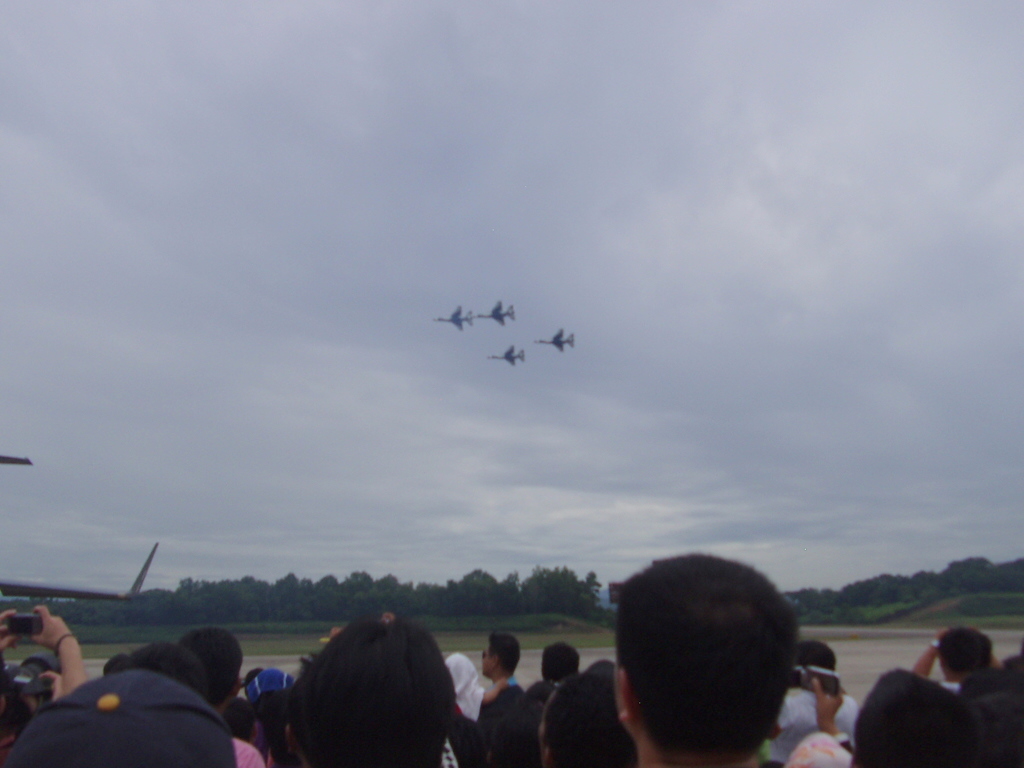In this photograph taken at an air show on an overcast day, the cloudy sky dominates the scene, providing a backdrop for four fighter jets flying in a tight, diamond-shaped formation, possibly Navy Blue Angels. Below, the foreground is filled with the backs of spectators' heads, some wearing hats and t-shirts, while others hold cameras or phones aloft to capture the moment. A flat area or runway extends at ground level, bordered by low rolling hills and a long row of trees in the distance, framing the spectacle in the sky.